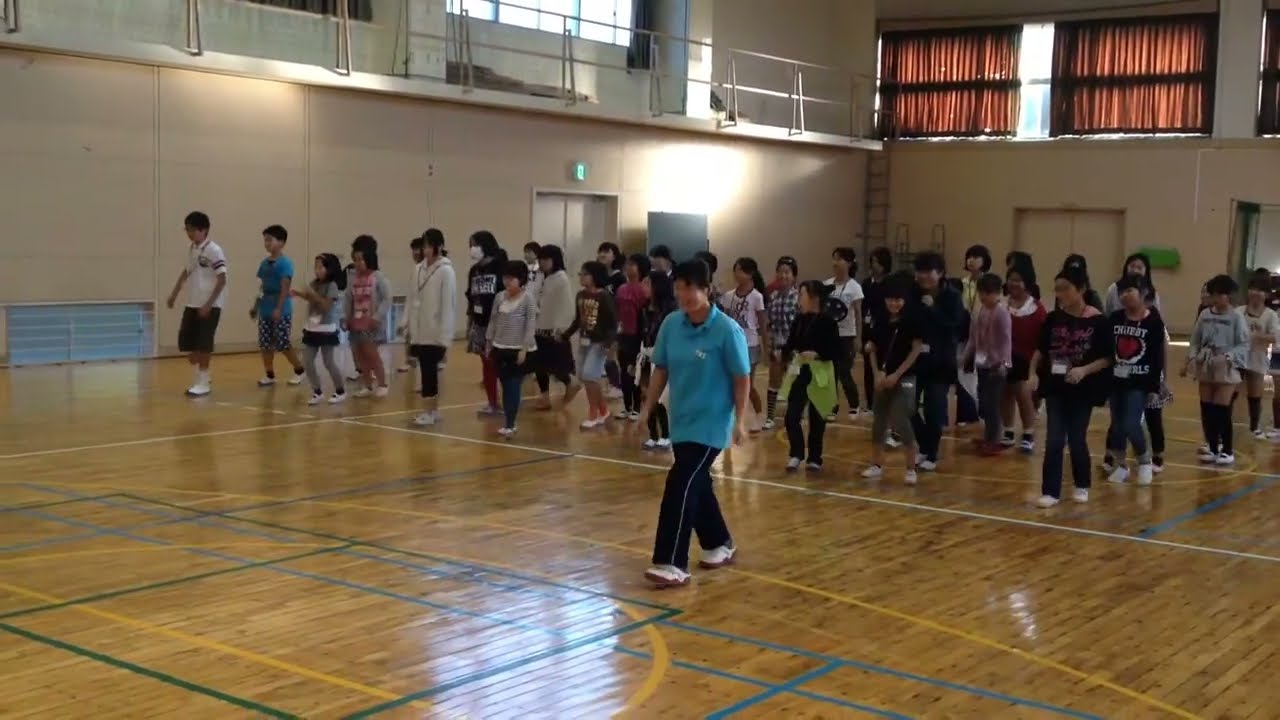In a brightly lit indoor school gymnasium, an Asian woman, possibly a teacher, stands at the forefront, wearing a blue shirt, black pants, and white sneakers. Her short hair complements her energetic stance as she leads a large group of students. Behind her, around twenty to thirty Asian students, estimated to be between eight to ten years old, are arranged loosely in rows on a shiny, polished basketball court marked with green and white lines. The students, dressed in various casual outfits including jeans and T-shirts, appear attentive, with some seemingly in the middle of an exercise or dance routine. Background details include a mezzanine with a railing, a white wall interspersed with windows covered by brown shades through which sunlight streams in, and a hint of a green light above what looks like an elevator door.